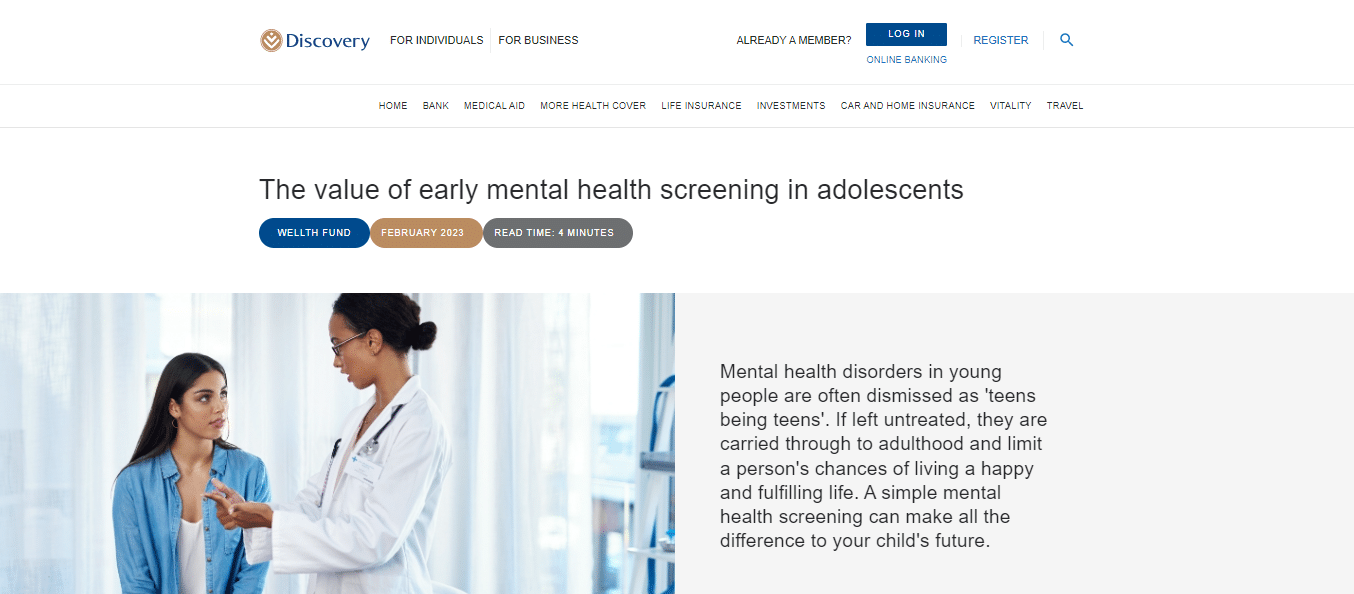**Screenshot from a Webpage Highlighting the Importance of Early Mental Health Screening in Adolescents**

The screenshot features a clean white background with various elements organized systematically. In the top-left corner, there is a logo accompanied by text in blue that reads "Discovery." Adjacent to the logo, black text displays navigation options: "For Individuals or Business," "Already a Member," "Login," "Online Banking," "Register," and "Search." A faint gray line separates this section from the main content below.

The next segment consists of a navigation bar with categories in black text: "Home," "Bank," "Medical Aid," "More Health Cover," "Life Insurance," "Investments," "Car and Home Insurance," "Vitality," and "Travel." This is followed by another faint gray line, beneath which is a headline in black text: "The Value of Early Mental Health Screening in Adolescents." Below the headline, there are three colored ovals indicating metadata: a blue oval labeled "Wealth Fund," a tan oval with "February 2023," and a gray oval reading "Read Time or Minutes."

On the left side of the screen, an image depicts a young woman with dark skin, long dark hair pulled into a bun, glasses, and a white lab coat with a stethoscope. She is speaking to a seated woman with tan skin and long dark hair, wearing a white shirt layered with a blue button-up shirt. The setting appears to be a hospital or clinic room.

To the right of this image, text discusses the issue of mental health disorders in young people:

"Mental Health Disorders in Young People are Often Dismissed as Teens Being Teens. If left untreated, they are carried through to adulthood and limit a person's chances of living a happy and fulfilling life. A simple mental health screening can make all the difference to your child's future."